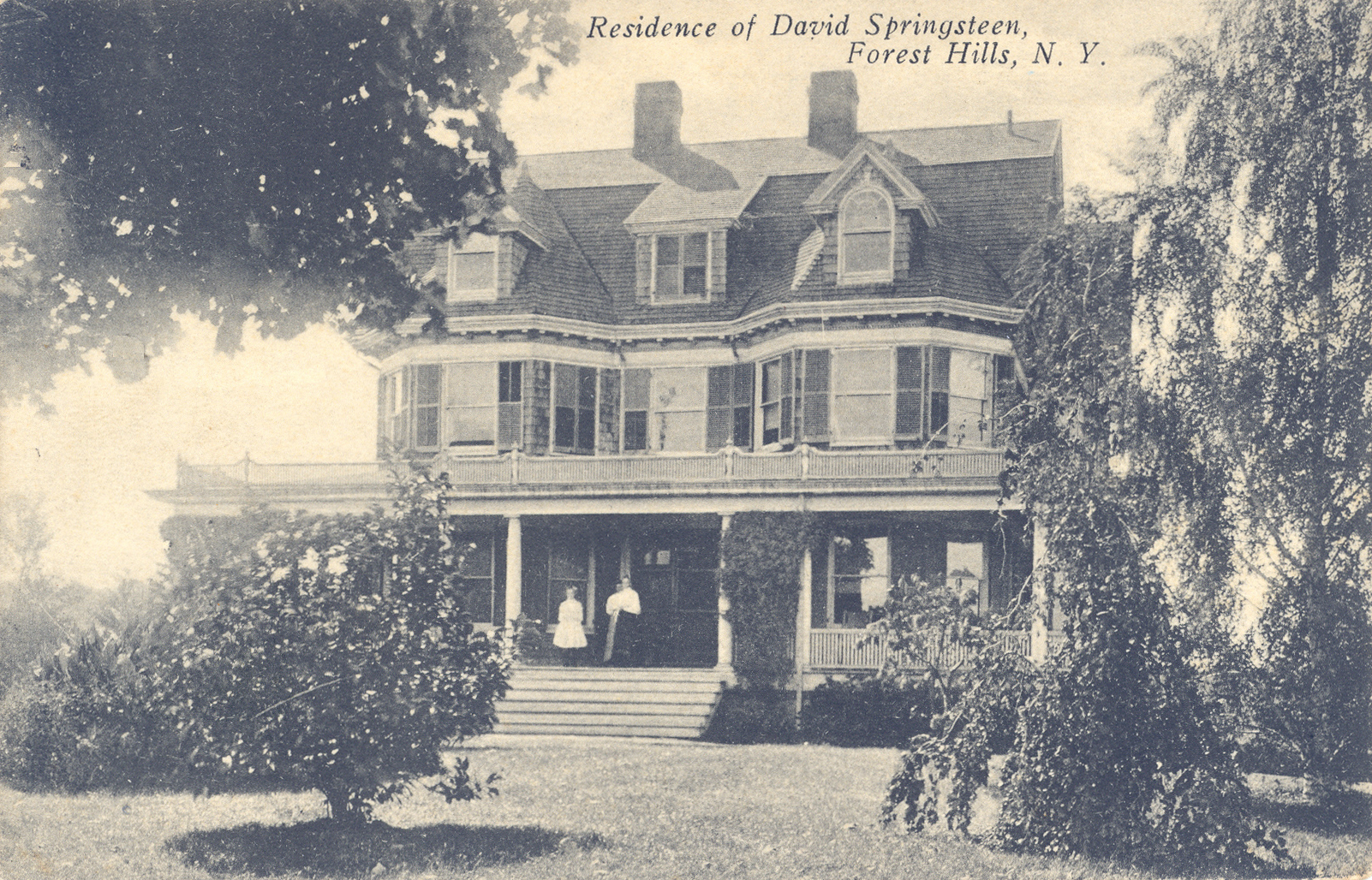This old black-and-white photograph, tinged with sepia tones, depicts a grand, three-story Victorian-era house identified at the top of the image as the residence of David Springsteen in Forest Hills, New York. The house, resembling a dollhouse with its intricate design, features numerous gables and large bay windows on the upper floors. A spacious wraparound veranda adorned with a few steps leads up to the grand entrance. Standing on the veranda are two or three individuals, one distinctly female in a simple, white, old-fashioned dress, and another figure possibly male or female, dressed in a white shirt and dark, plumed-out skirt holding a stick. The front yard is lush with trees, including one draped with hanging moss, adding to the serene, historic ambiance. The photograph, likely from the early 1900s, captures not just the architectural charm of the palatial home but also a glimpse into the period through the fashion and style of the individuals present.